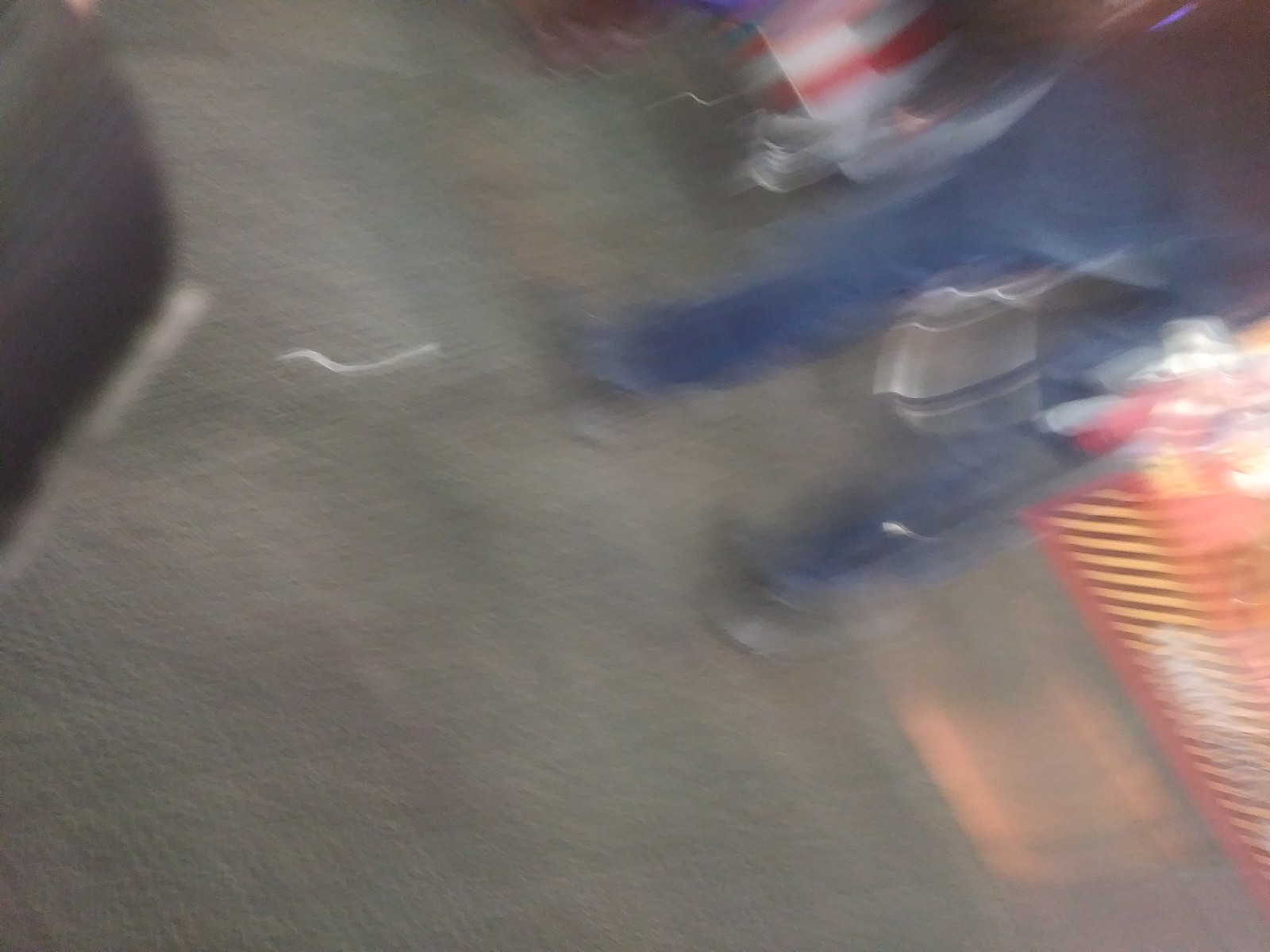The image is a very blurry, seemingly rotated photograph that captures the bottom half of a man wearing blue jeans and tennis shoes. The man appears to be carrying a couple of bags, one of which is gray with navy blue stripes. The background shows a floor that looks like pavement, alongside a table with red and white stripes. To the left side of the man, there is a chair. Additional elements in the image include a tablecloth to the right that features red, yellow, and brown colors, as well as a flat piece of metal in front of the person. The image also shows a backdrop that resembles a little wall or marketplace booths, predominantly red with some designs. The photograph lacks textual details, making it challenging to discern subtle features due to its blurriness.